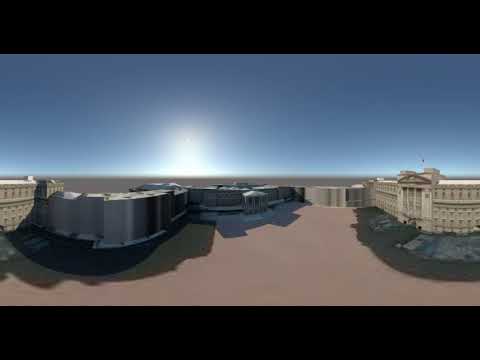The image showcases a 360-degree panoramic scene with a light brown, possibly cement ground flanked by thick, black rectangular borders at the top and bottom. At the center of the image, there is a vast, clear blue sky with a bright, blurry white sun positioned slightly to the left but close to the middle. The skyline features a continuous stretch of interconnected buildings. Dominating the right side of the image is a tall, classical white building, possibly historical, with multi-story pillars and intricate detailing. This building curves towards the center and merges seamlessly with a simpler, gray-edged building. On the far left, the architectural flow continues with a more modern, multi-story structure with numerous windows and repeating patterns. The background is filled with blurred, featureless gray structures resembling government buildings, extending to a perfectly straight horizon. This composite scene merges classical and modern architectural styles, giving an impression of a historical site with modern additions, under a pristine, clear sky.